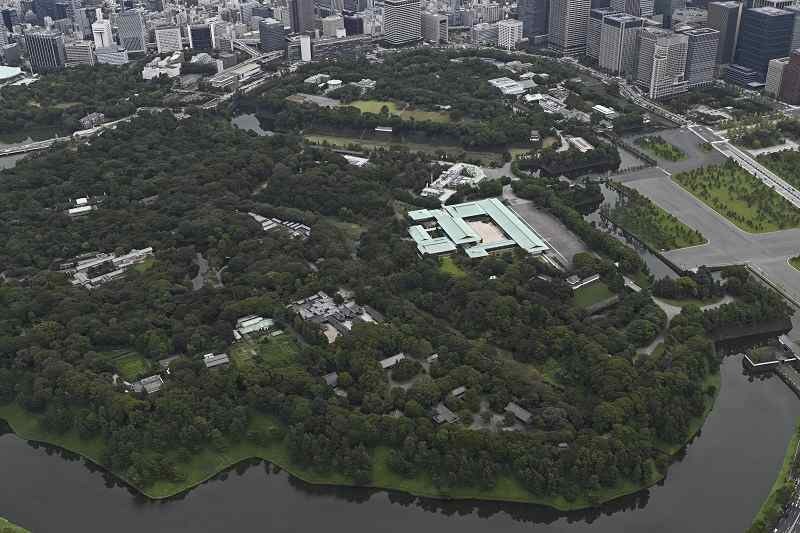This aerial image likely depicts a city, offering a rich view of diverse elements. Dominating the foreground, a dense, lush patch of dark green trees is intermittently dotted with smaller buildings. This verdant area is juxtaposed against a dark, murky body of water which could be either a river or a lake, stretching horizontally across the lower portion of the image. Toward the top, forming the distant background, a sliver of towering, dark-colored skyscrapers stands, tinged with blues, blacks, and occasional white accents. Among the trees, pathways and roads weave through, leading to various buildings. Notably, to the far right, a possible factory or industrial site can be seen, with accompanying highways and roads faintly visible. The image is taken during the day, predominantly showcasing shades of green, black, and white, providing a stark contrast between the natural and urban elements of the cityscape.